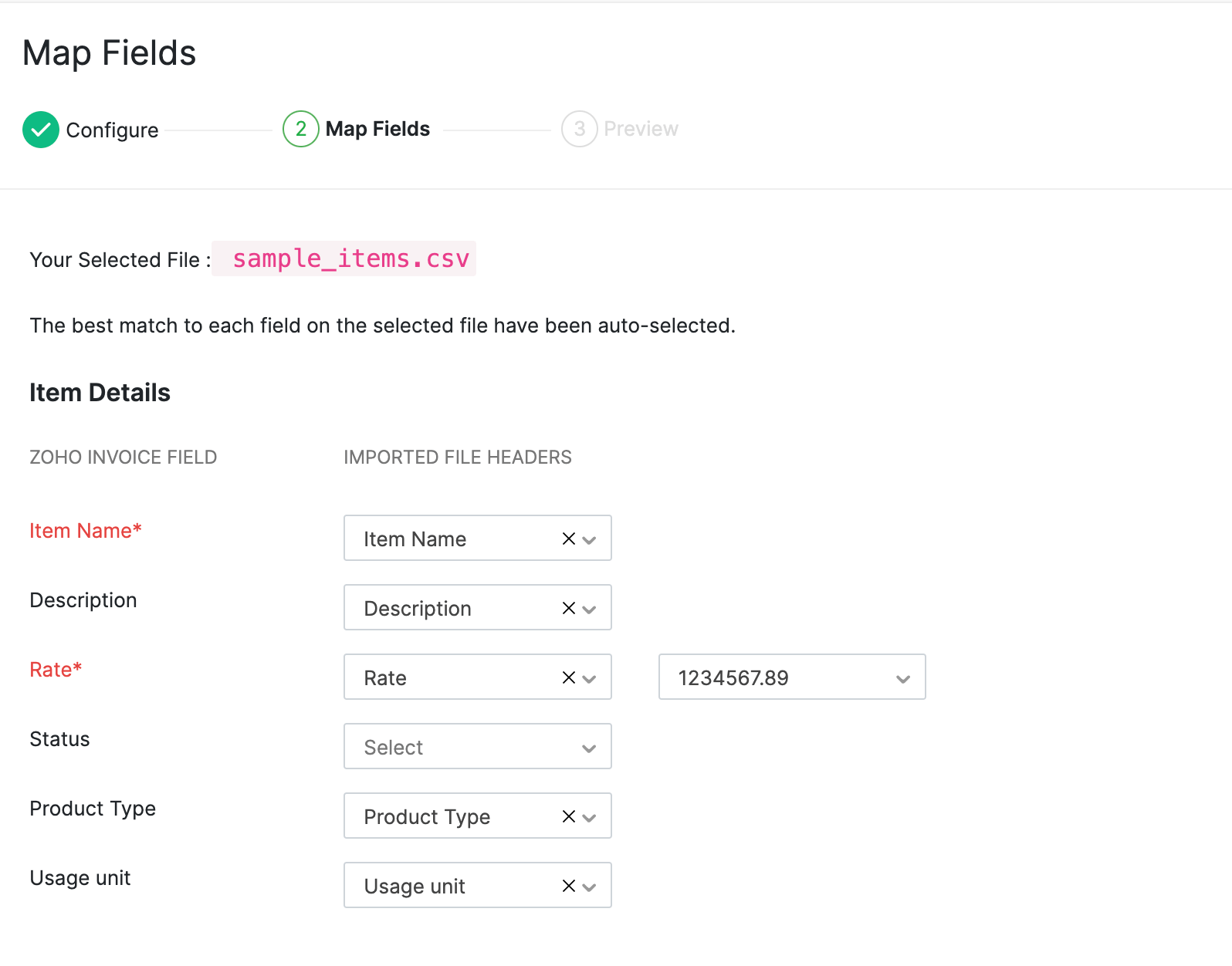In this screenshot taken from a website about mapping fields, several key elements are displayed clearly. At the top-right corner, the text "Map Fields" is prominently written in black. Just below this title, there is a green circular icon featuring a white check mark. Adjacent to this icon, towards the left, the black text "Configure" is visible. Moving further to the right, almost towards the center of the image, there is another circular shape showcasing a green number "2" in its middle, with the adjacent black text reading "Map Fields."

Below this header, in smaller black text, the phrase "Your selected file:" can be seen, followed by "sample_items.csv" written in bright pink. Beneath this, a notification in black informs that the best match to each field in the selected file has been auto-selected.

The screenshot continues with a bold black heading "Item Details," and below it, in medium gray text, it reads "Some invoice fields." To the right of this, "Imported Field Headers" is indicated. Below, in a table format, "Item Name" is written in red with an asterisk, followed by dropdown options for "Description," "Description X," "Rate," "Status," "Product Type," and "Usage Unit" each accompanied by a downward pointing arrow inside a square. 

The background of the webpage is predominantly white, providing a clean and clear interface for users to interact with.